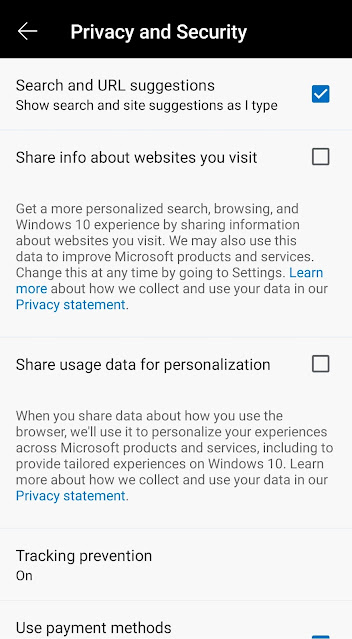The image is a screenshot taken from a cell phone displaying a "Privacy and Security" settings menu. At the top of the screen, there is a black header with a white left-pointing arrow. The header text, in white letters, reads "Privacy and Security." Below it, in smaller black print, the first setting is labeled "Search and URL Suggestions." Next to this label, a checkbox is marked with a blue check, indicating that the option is enabled. This setting also includes a subtext explaining "Show search and site suggestions as I type."

Further down, another setting is titled "Share info about websites you visit." This option includes a paragraph and an empty checkbox, indicating it is not enabled. Below this, there's a setting called "Share usage data for personalization," accompanied by another explanatory paragraph. Both this paragraph and the preceding one contain the term "privacy statement" highlighted in blue, presumably linking to additional information. The checkbox next to this setting is also unchecked.

Towards the bottom of the screen, the text "Tracking prevention" is shown as activated with the word "On." Additionally, there is an option labeled "Use payment methods." The screenshot comprehensively captures the intricate details of various privacy settings available on the device.